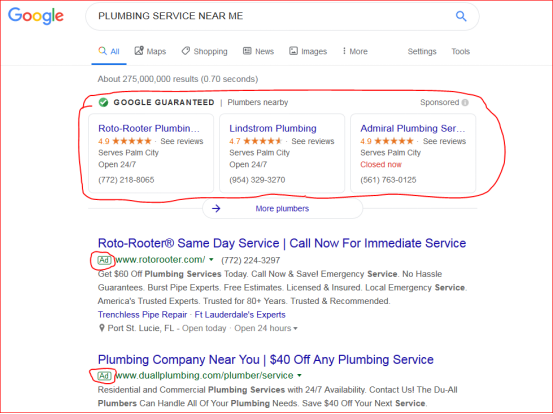The image displays a Google search results page for "plumbing services near me" with Google's logo situated in the upper left corner, all enclosed within a thin red outline. The results summary indicates there are approximately 275 million results, retrieved in 0.7 seconds. At the top of the page, the search options include "All," "Maps," "Shopping," "News," "Images," "More," "Settings," and "Tools."

Prominently featured at the top of the search results is a section labeled "Google Guaranteed," which is hand-circled with an uneven red line, indicating a paid advertisement. It features three primary listings for plumbing services:

1. **Roto-Rooter Plumbing**
   - Rating: 4.9 stars
   - Call to action: See reviews
   - Location: Serves Palm City
   - Availability: Open 24/7
   - Contact: 772-218-8065

2. **Lindstrom Plumbing**
   - Rating: 4.7 stars
   - Call to action: See reviews
   - Location: Serves Palm City
   - Availability: Open 24/7
   - Contact: 8945-329-3270

3. **Admiral Plumbing**
   - Rating: 4.9 stars
   - Call to action: See reviews
   - Location: Serves Palm City
   - Availability: Closed now (highlighted in red)
   - Contact: 561-763-0125

Below these, there are two additional listings marked as ads, each circled in red.